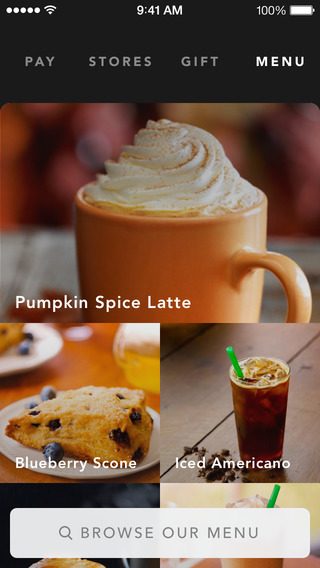Screenshot featuring a festive pumpkin spice latte. At the top of the image, there's a partially visible black rectangle with illegible text. The background is a combination of burgundy, gray, and white hues. In the center, a vibrant pumpkin-colored coffee cup holds a pumpkin spice latte crowned with a swirl of whipped cream. The whipped cream is garnished with a sprinkling of pumpkin-colored spices. Below the coffee cup, the words "Pumpkin Spice Latte" are prominently displayed in white text. To the left of the cup, a white plate showcases a delicious blueberry scone. To the right, an iced Americano sits in a clear cup, marked by a green straw. At the bottom of the image, a white triangle with a magnifying glass icon and the gray text "Browse Our Menu" invites viewers to explore more options.